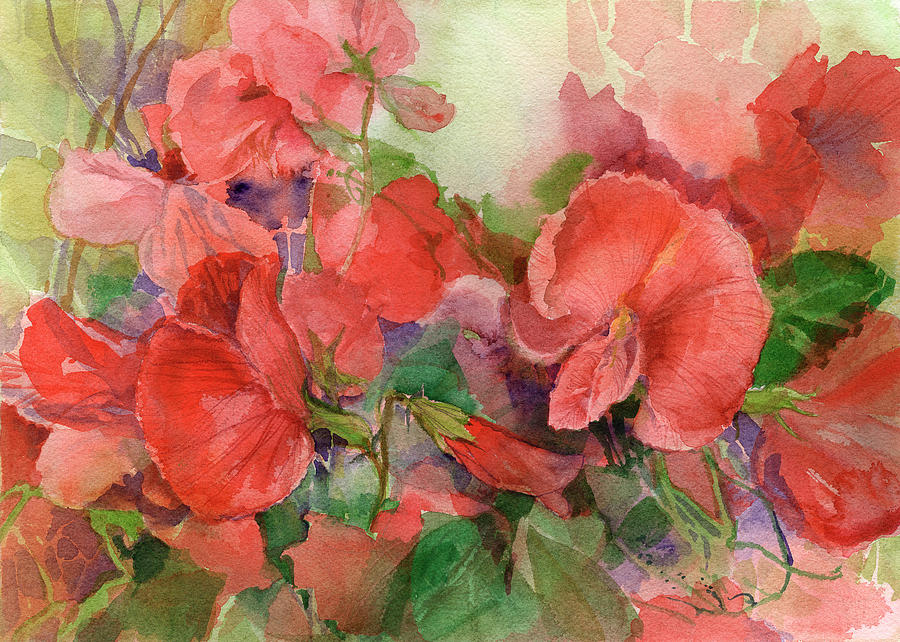This is a slightly abstract painting, predominantly featuring an array of flower petals and leaves. The flowers, varying in shades of red and pink, are surrounded by green foliage. At the bottom, green stems and leaves emerge, short yet abundant. In the middle section, the flower petals become more prominent, transitioning from darker red flowers on the left to lighter red and pink hues in the center and right. The upper part of the painting continues this color gradient, with the top left corner showcasing pink flowers amidst light green stems and plants. The upper right follows with a mix of red, light red, and pink flowers. Some flowers are fully bloomed, displaying rich red tones, while others appear as buds. The style resembles watercolor over pencil on canvas, creating a beautifully detailed representation that might evoke the feeling of a garden or a bouquet of flowers.